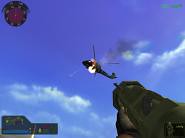In this detailed screenshot from a video game, the perspective is angled upwards, capturing a vivid, bright blue sky adorned with realistic, fluffy white clouds that impressively mirror real-life graphics. Dominating the center of the image is an action-packed scene featuring a helicopter enshrouded in billowing grey smoke and ablaze with orange flames, evidence of its recent explosion. In the bottom right corner, the player’s character is visible, wielding a black weapon while adorned with protective gloves, emphasizing their active engagement in the scenario. Additionally, the game's interface elements are partially visible; a circular compass is located in the top left corner, providing navigational information, while the bottom left corner includes parts of the character's HUD, possibly indicating their status or available ammunition.